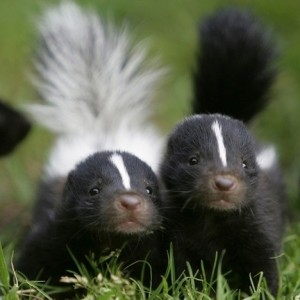This color photograph, taken in a realistic representational style and presented in a square format, features two young skunks standing side by side in a natural setting of green grass. The skunks, with their black fur adorned with distinctive white stripes, face slightly up towards the top right, offering a front view to the viewer. Both have small, beady black eyes, fluffy tails, and beige-colored noses and mouth areas, framed by whisker-like hairs.

The one on the left sports a prominent white stripe running from its forehead down its back, widening significantly near the rump and extending into a full, bushy white tail. In contrast, the skunk on the right has a thinner white stripe along its side and a larger but less wide, all-white tail. While both skunks lack visible ears, they exhibit a somewhat identical facial structure, with the one on the right appearing slightly more mature and having a more elongated face. The background of the image is out of focus, emphasizing the detailed depiction of the skunks in their grassy environment.